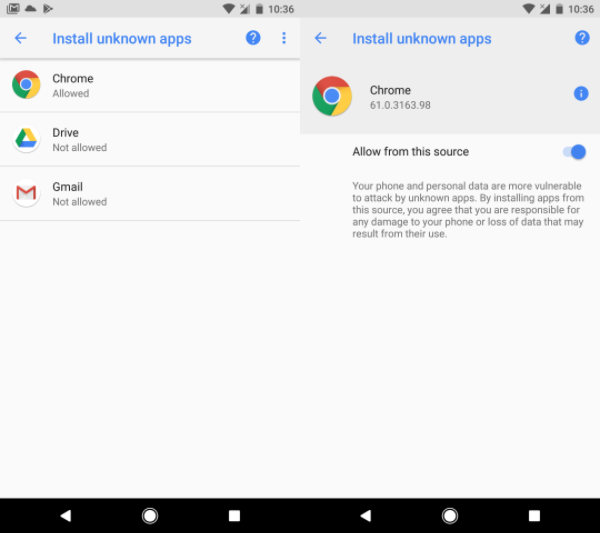A screenshot of a Google Chrome web page is displayed on a device. At the top of the screen is the menu bar, featuring symbols for battery life, reception, and the time, which reads 10:36. Directly beneath the menu bar, the heading "Install unknown apps" is visible, accompanied by a left-pointing arrow. Below this heading is a list of apps, starting with "Chrome," represented by the circular logo composed of red, yellow, green, and blue. Following "Chrome," there is "Drive" with its triangular logo and "Gmail."

Underneath each app name, there are relevant permissions listed: "Chrome is allowed," "Drive is not allowed," and "Gmail not allowed." "Chrome" appears to be highlighted. Below the highlighted "Chrome," there is a heading that reads "Allow from this source." Under this heading, there is a warning message: "Your phone and personal data are more vulnerable to attack by unknown apps. By installing apps from this source, you agree that you are responsible for any damage to your phone or loss of data that may result from their use."

At the very bottom of the screen, navigation symbols are present: a triangle pointing to the left, a circle, and a square, indicating options to navigate back, and possibly other functions.